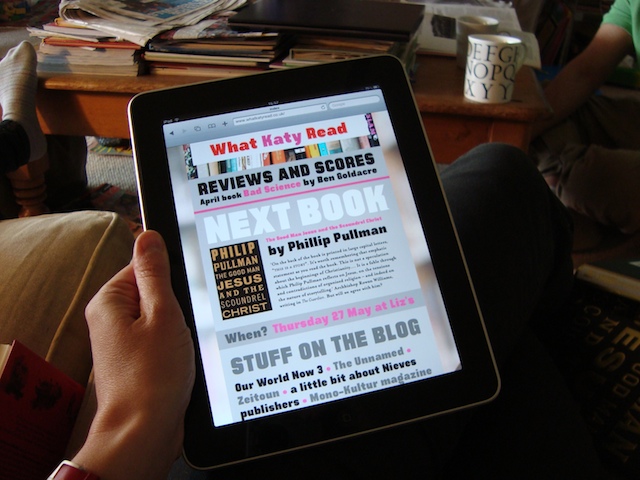In this detailed image, a person is holding an old iPad, identifiable by its chunky borders and silver edge, likely one of the first models. The iPad's screen features a webpage titled "What Katie Read." Within the webpage, there are several sections including a review for the book "Bad Science" by Ben Goldacre and an upcoming feature on "The Good Man Jesus and the Scoundrel Christ" by Philip Pullman, scheduled for Thursday, May 27. Additional blog sections preview various topics like "Liz's Stuff on the Blog," "Our World Now Three," "The Unnamed Z-Tune," and "A Little Bit About Neves Publishers." The person appears to be sitting on a brown couch, and in the background, there's a desk or coffee table cluttered with newspapers, books, and a coffee mug featuring the alphabet. The setting resembles a communal space, possibly a study room, coffee shop, or a living room, with other people present in the vicinity.